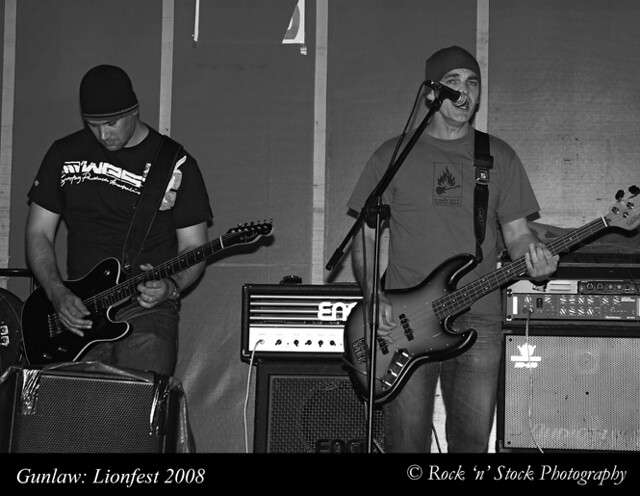This black-and-white photograph captures a candid moment of two men performing on stage at Gun Law Lion Fest 2008, as indicated by the white text on a black banner at the bottom of the image, which also credits Rock ‘N Stock Photography. The man on the left, wearing a black beanie, a black t-shirt with white writing on the front, and jeans, strums a black electric guitar. In front of him is an amplifier, part of the various musical equipment and cords arranged on stage. The man on the right, donning a lighter-colored beanie and a dark gray shirt with jeans, is singing into a microphone while playing a light-colored electric bass guitar with a black outline. He stands directly before two large amplifiers, adding to the array of recording equipment visible behind them.